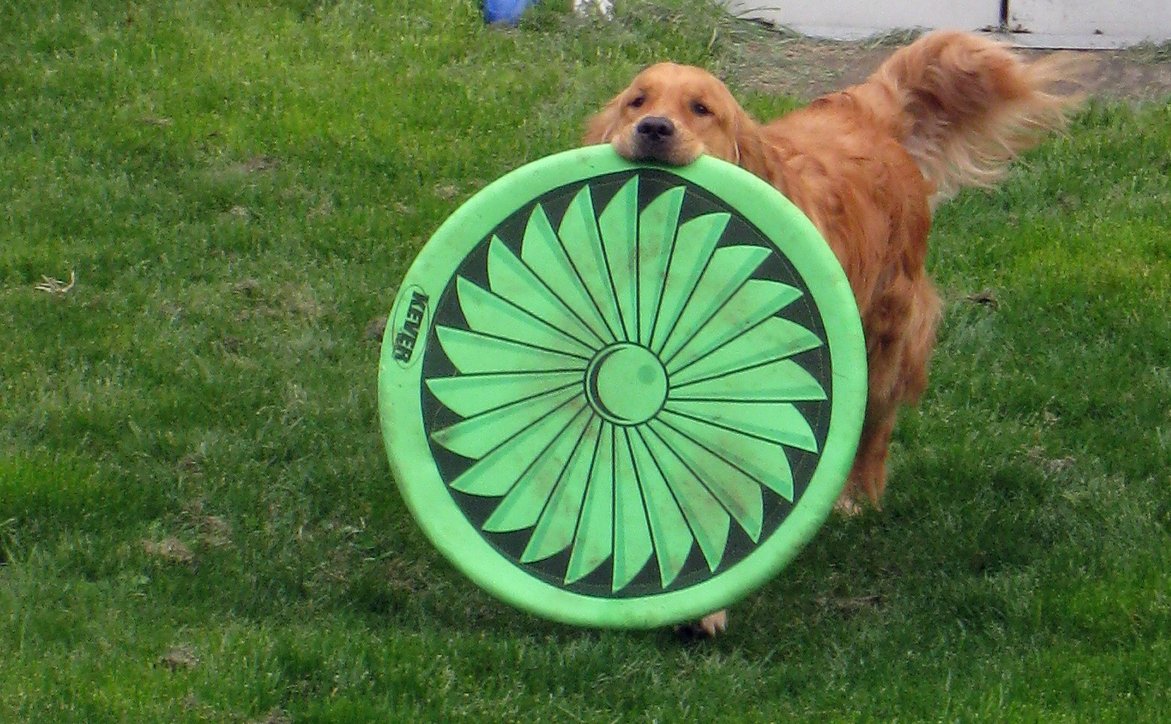In this captivating photograph, a beautiful golden retriever with a light reddish-brown coat and fluffy tail stands proudly on a lush grassy area adorned with varying shades of green. The dog’s expressive brown-black eyes, black nose, and a hint of black fur beneath his nose add to his charming appearance. Clutched in his mouth is an enormous pale green frisbee, so large it nearly matches the size of the dog himself. The frisbee features a flowered fan decoration in the middle, with a green and black pattern that has become dingy from vigorous play. The edge of the frisbee bears partially visible letters, possibly spelling "Never" or "K-E-V-E-R." In the background, beyond the vibrant grass, there's a hint of a sandy beach leading to a body of water where someone is standing. The dog appears dry, with his tail raised and ears flopped down, eagerly carrying his treasured frisbee, perhaps from a recent fun-filled romp by the waterside.